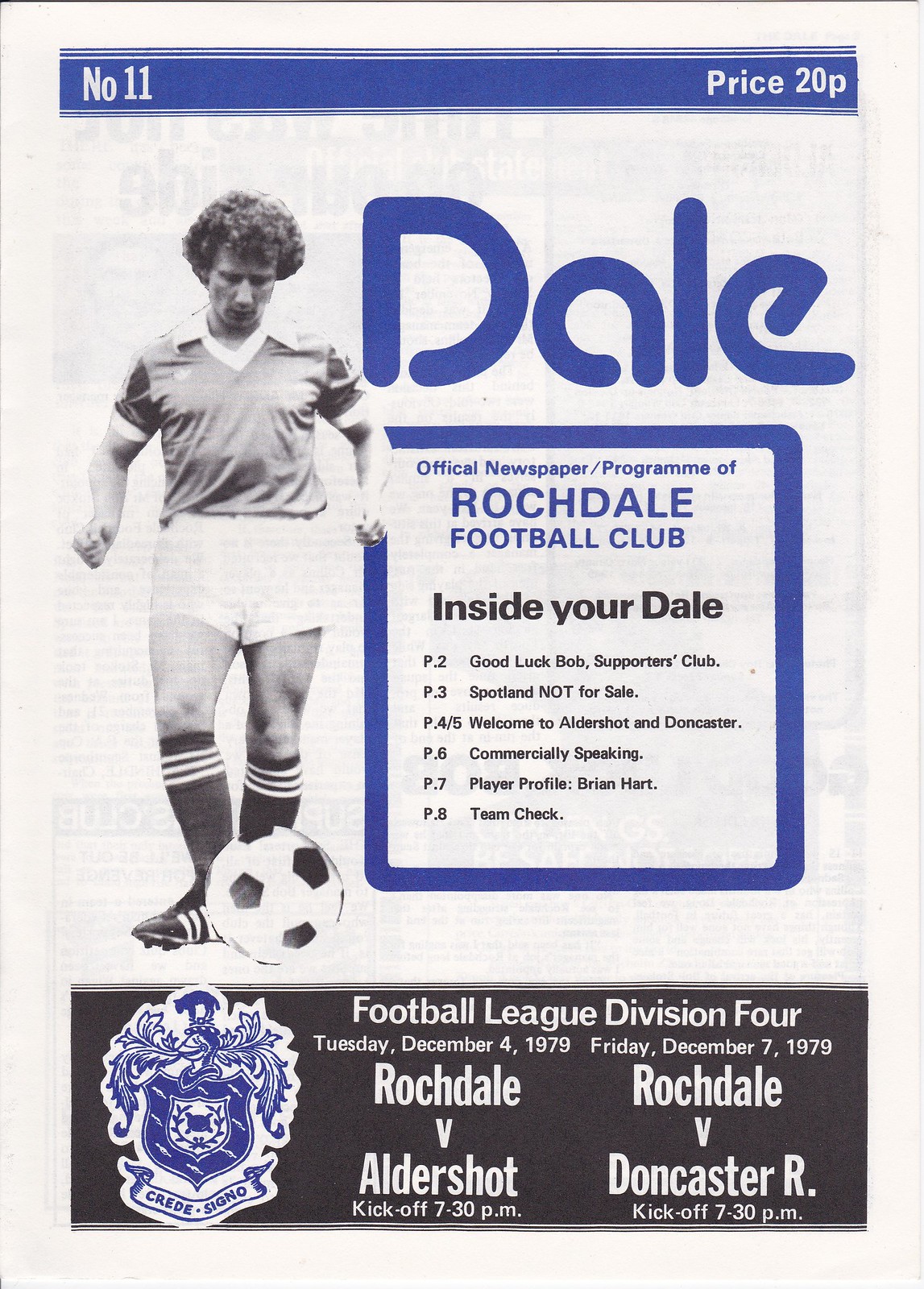The image depicts a vintage football program believed to be from Rochdale Football Club. Dominating the entirety of the image is a white background program with a blue horizontal strip at the top that has white borders. On the left side of this strip, in white lettering, it says "NO. 11" and on the right side, "PRICE 20p."

Below this strip, on the left side, we see a black-and-white picture of a football player with curly hair, wearing a collared jersey, white shorts, black leggings, and black shoes. The player is captured mid-kick with a soccer ball positioned at his feet. 

To the right of the player, the word "D-A-L-E" is prominently displayed in large blue letters. Below this title, a blue-bordered box with a white background contains several sections of text. The text in blue reads, "Official newspaper/program of Rochdale Football Club." In black, it details the contents of the program: "Inside Your Dale (Page 2)," "Good Luck, Bob (Supporters Club, Page 3)," "Spotland Not for Sale (Page 4 & 5)," "Welcome to Aldershot in Doncaster (Page 6)," "Commercially Speaking (Page 7)," "Player Profile: Brian Hart (Page 8)," and "Team Check."

At the bottom of the image, there is a black rectangle with white text that indicates the match details. On the left side, there is a shield-like logo with floral designs featuring a cat and a ribbon on top that reads "GREAT," and next to it, the match schedule is printed: "FOOTBALL LEAGUE DIVISION FOUR - Tuesday, December 4, 1979: Rochdale vs. Aldershot (Kick-off 7:30 PM), and Friday, December 7, 1979: Rochdale vs. Doncaster R (Kick-off 7:30 PM)."